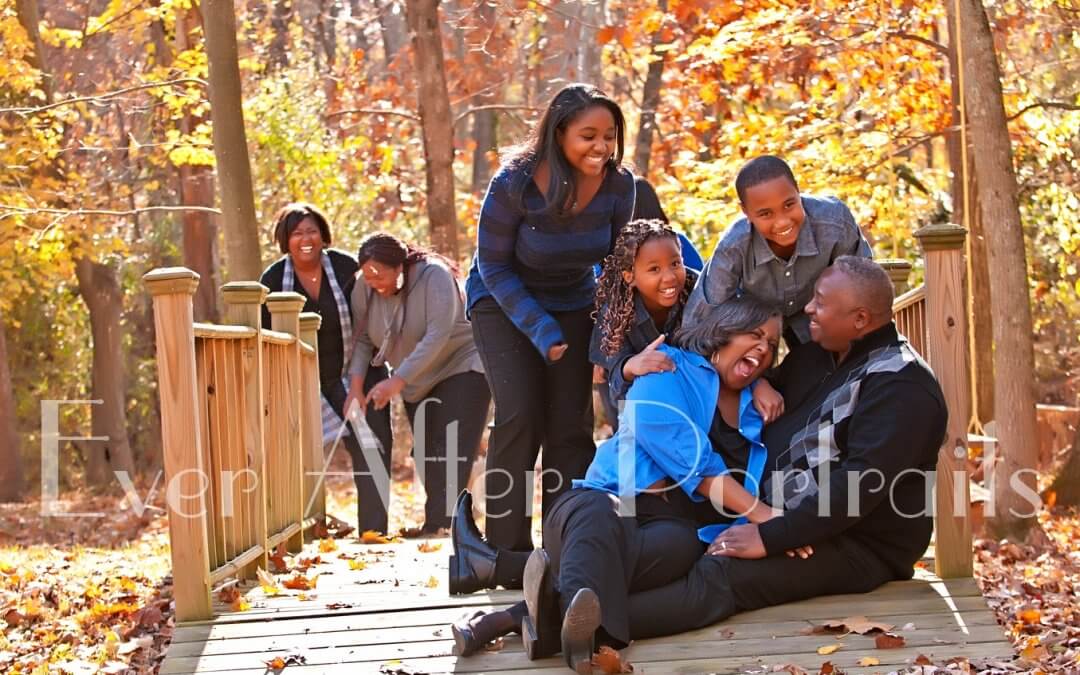This horizontal rectangular photograph is an advertisement for Ever After Portraits, featuring a joyful African American family in a picturesque fall setting. The family, consisting of parents and their three children, is gathered on a wooden bridge in a wooded park. The bridge, constructed from light-colored wood with railings, sits amidst golden autumn leaves. Both the mother and father, with the father sporting gray hair, sit on the bridge, the mother’s legs draped over the father’s in a playful, affectionate manner. The scene is filled with laughter and smiles from everyone, including the three children standing or leaning over the bridge railings behind them. The sun filters through the colorful foliage, casting a warm glow on the family, amplifying the vibrant autumn hues. The text "Ever After Portraits" overlays the image in faint white, blending seamlessly with the serene, happy atmosphere of the scene.